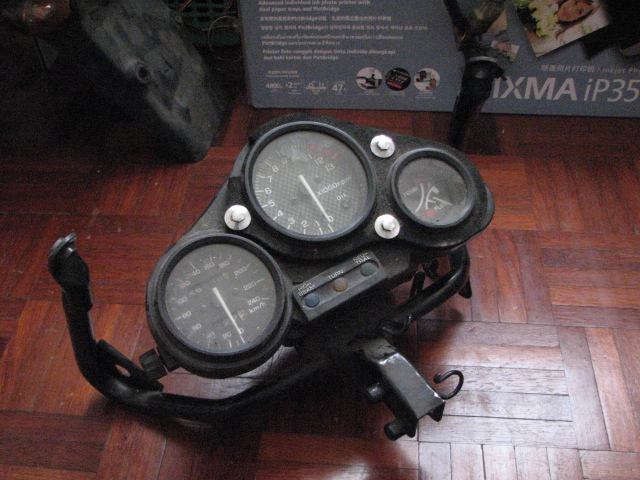The image captures the interior of a home, possibly a garage or living room, with distinct reddish-brown wood panel flooring. The floor, composed of square panels, adds a rustic charm to the setting. At the center of the image, there are three black speedometers, which seem to have been dismantled from a motorcycle and meticulously arranged on the floor. Behind the speedometers, a PIXMA IP35 printer box is visible, indicating some ongoing activity that involves both technology and machinery. In the upper left corner, shadows obscure what appears to be another component, likely related to the motorcycle. The detailed arrangement and the juxtaposition of the objects create an intriguing and intricate scene.